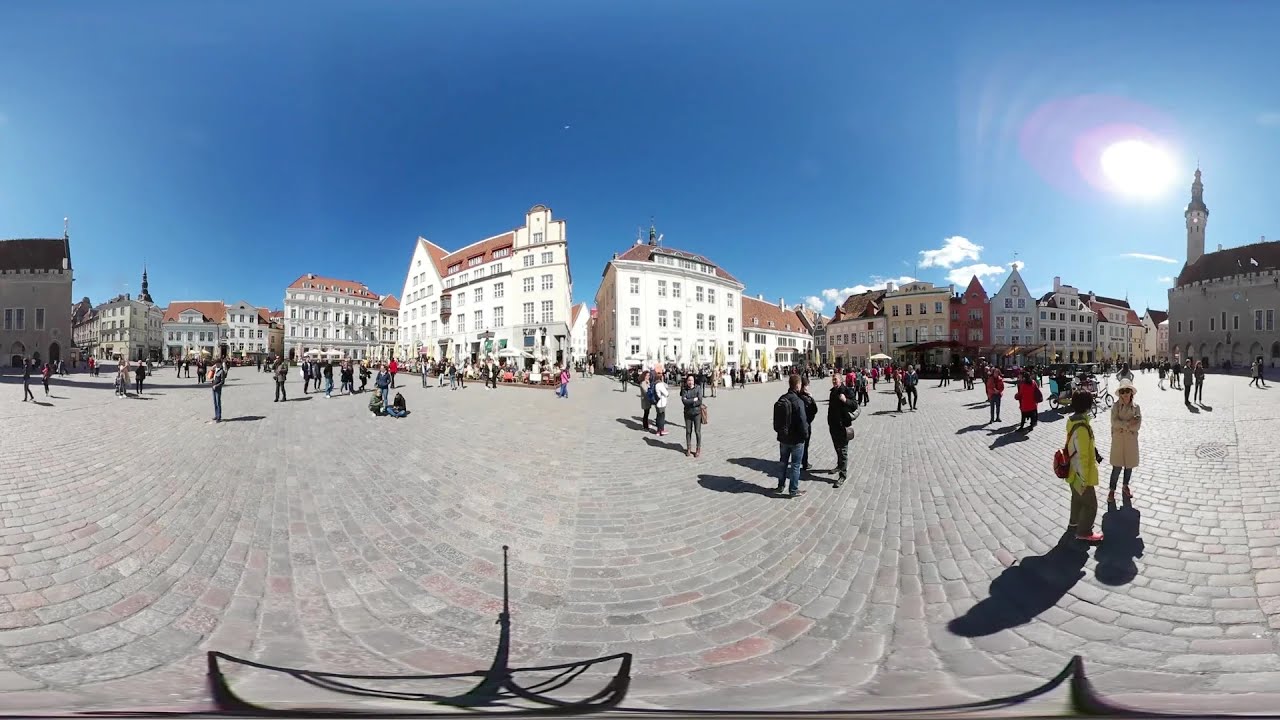This panoramic image captures a bustling courtyard area in a tourist town, with a vivid blue sky and sparse clouds overhead. The ground is a widespread expanse of flagstone and brick, weaving a textured, gray foreground. Clustered throughout the expansive open area are people milling around in small groups, conversing and walking. Dominating the scene are numerous multi-story buildings with slanted roofs, varying in hues from white and beige to brown and brick red. Each building has up to three stories with glass doors set in wooden frames. The architectural centerpiece at the right edge of the picture is a church with a dark roof and a prominent tower. The bright, yellow sun shines overhead, creating sharp shadows and a slight image distortion due to its glare. A distinct road runs between the closely grouped buildings in the center, leading towards different streets branching away in the distance. The overall scene is lively and vibrant, with the clear, sunny weather adding to the picturesque quality of the town.